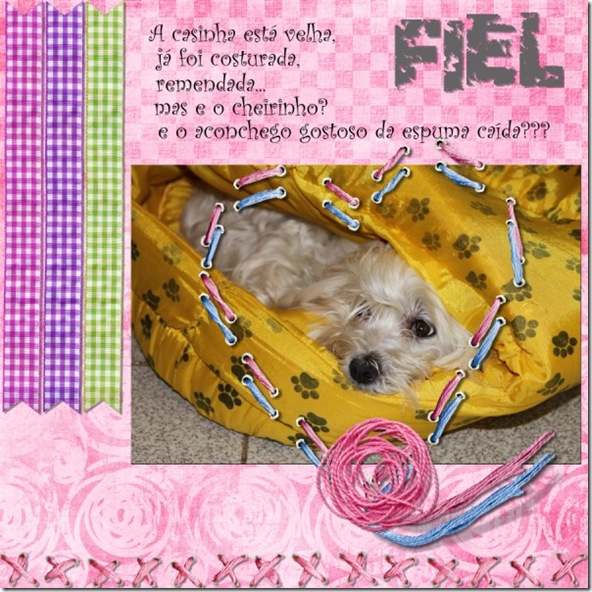This image showcases a meticulously crafted collage with rich details centered around a white, furry dog comfortably nestled in a pet bed that resembles a bag or purse. The dog, which exudes an air of contentment, is placed prominently in the center of the collage against the backdrop of a tile floor. The photo of the dog is encased within an elaborate, graphic border predominantly painted in shades of pink, alongside other hues such as purple, green, blue, and white. This border features intricate floral patterns and text in a foreign language, potentially Portuguese, adding an exotic touch to the composition.

Enhancing the collage are three checkerboard ribbons in pink, purple, and green, which drape from the top left side of the image. These ribbons contribute a playful, decorative flair. Below the dog's picture, there's a pink flower graphic with little "X" motifs, and a heart-shaped ribbon encapsulates the dog's image, lending a sweet, affectionate ambiance. The entire ensemble appears to blend themes of fabric, sewing, and possibly baby decor, intertwining soft textures and cozy elements in a warm, indoor setting.